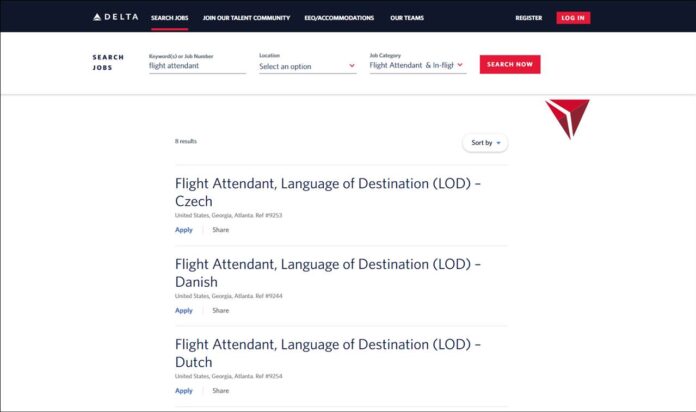The webpage appears to be Delta's job application platform, though the resolution is notably poor. At the top, there's a black strip featuring the Delta logo on the left, accompanied by a navigation menu offering options such as "Search Jobs," "Join Our Talent Community," "EEO Accommodations," and "Our Teams." On the right side of this strip, there is a "Register" button and a "Login" button, both in red with white font.

Below, there is a prominent search section, starting with the "Search Jobs" heading. Here, users can narrow down their search by selecting options from dropdown menus labeled "Location" and "Category," each featuring "Flight Attendant" and "In-flight" choices, respectively. To initiate the search, there's a "Search Now" button in red with white font.

Following a gray divider line, the results display begins, listing eight job matches. Each listing provides job details, starting with "Flight Attendant, Language of Destination (LOD): Check" for the first listing, which is located in Atlanta, Georgia, USA. There's also an unreadable reference number. Options to "Apply" (in blue) and "Share" (in gray) are available. Above the listings, there's a sorting option, "Sort By," with a dropdown menu for users to organize the results.

The second listing follows a similar format: "Flight Attendant, Language of Destination (LOD): Danish," located in Atlanta, Georgia, USA, again with an unreadable reference number, accompanied by "Apply" (in blue) and "Share" (in gray) options. The section concludes with a gray line separating the subsequent listings.